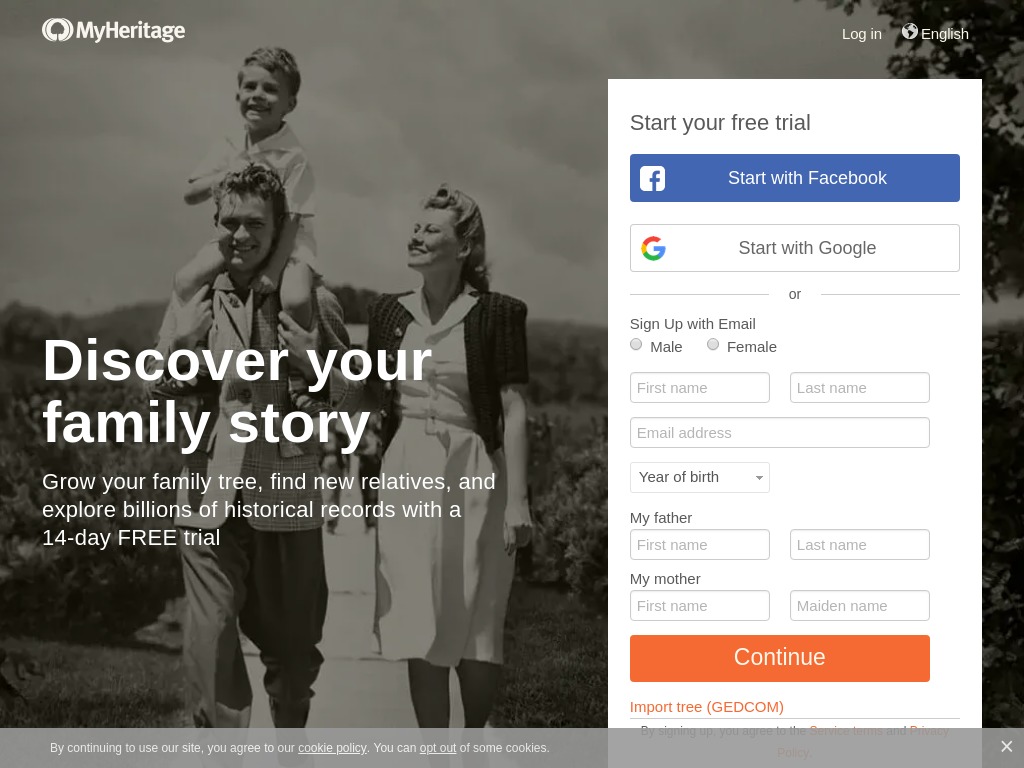This advertisement for MyHeritage, akin to Ancestry, features their logo—a white circle with a stylized, trimmed tree resembling a mushroom—prominently displayed at the top. On the right side of the page, there are options to log in and a language setting indicating "English."

The central message, "Discover your family story," is highlighted on the left in a black-and-white photograph. The image depicts a family scene from the late 1940s to early 1950s. A nostalgic portrayal, it shows a father carrying his child on his shoulders, while the mother, donned in a belted dress and a vintage hairstyle commonly seen in that era, smiles beside them as they walk down a sidewalk. This setting evokes a post-World War II ambiance, around 1947 or 1948.

Below the photograph, a tagline reads: "Grow your family tree, find new relatives, and explore billions of historical records with a 14-day free trial."

To the right, the ad prompts viewers to "Start your free trial" with two prominently displayed buttons: a blue rectangle labeled "Start with Facebook" and a white rectangle labeled "Start with Google." Alternatively, users can sign up with their email, with smaller text indicating this option. The form requests details such as gender, first and last names, email address, year of birth, father's name, and mother's maiden name. The call-to-action button "Continue" is the next step in the signup process.